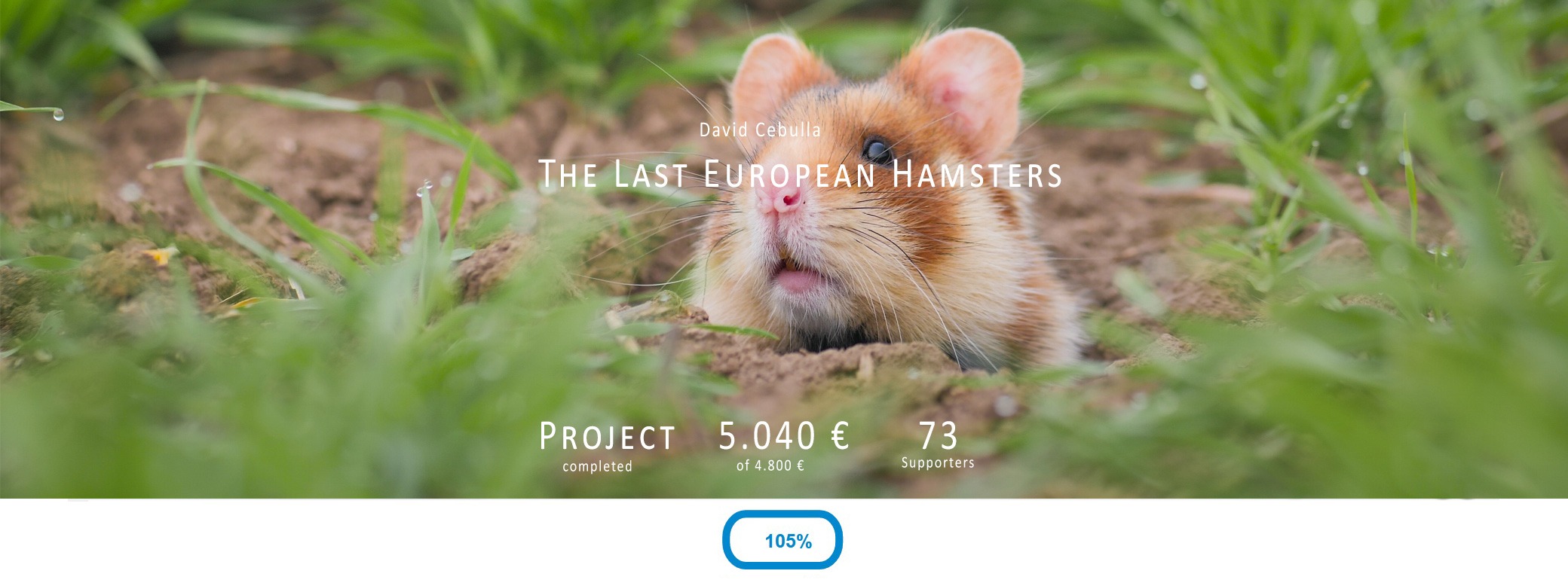The image is a vibrant outdoor graphic capturing a ground-level scene. The foreground is dominated by rich, kelly-green grass, visibly dotted with glistening water droplets, extending seamlessly to the background and framing the central subject on all sides. Emerging from a small burrow in the earth is the head of a European hamster, identified in the caption.

The hamster displays a striking tricolored fur pattern: black dominates the top of its head, transitioning to a sorrel, orangey-brown hue, and finally a light tan. Its pink nose is slightly lifted, and its mouth is slightly open, revealing pink lips and a white chin. The animal's black and white whiskers frame its face, and its round, brown eyes are clearly visible. The hamster’s ears are small and rounded, and the animal is angled to the right, showing more of its left side.

Overlaid text provides context and additional information. In white print near the top, the name “David Sebula” (C-E-B-U-L-L-A) is prominently displayed. Below this, in bold capital letters, the text reads “THE LAST EUROPEAN HAMSTERS.” Toward the bottom of the graphic, the project's completion status is summarized: “Project Completed.” The accompanying fundraising data indicates a goal of 5,040 pounds, with 4,800 pounds raised by 73 supporters. A white box at the bottom, outlined in blue, highlights the achievement in blue text: “105%.”